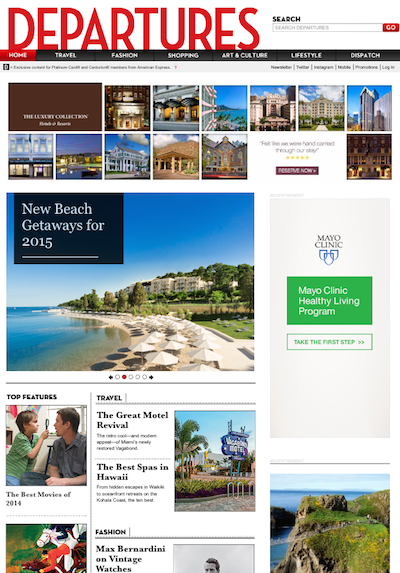Screenshot of a website, likely a news or travel website titled "Departures," as indicated by the prominent, bold, red text on the top left. The site's layout features a search bar on the top right, accompanied by a red "Go" button. A navigation bar at the top showcases various tabs: Home, Travel, Fashion, Shopping, Art and Culture, Lifestyle, and Dispatch - with the current selection highlighted in red, signifying the 'Home' tab is active.

Dominating the middle of the page is a large, sunny beach image. In the top left corner of this image, a black box contains the text "New Beach Getaways for 2015," indicating the screenshot's age. Below the picture, on the bottom left, are several feature articles. One article titled "The Best Movies of 2014" shows a boy in a green shirt holding a magnifying glass up to his presumed father, with both of them making eye contact. Adjacent to these features, on the right, are additional articles titled "The Great Motel Revival" and "The Best Spas in Hawaii."